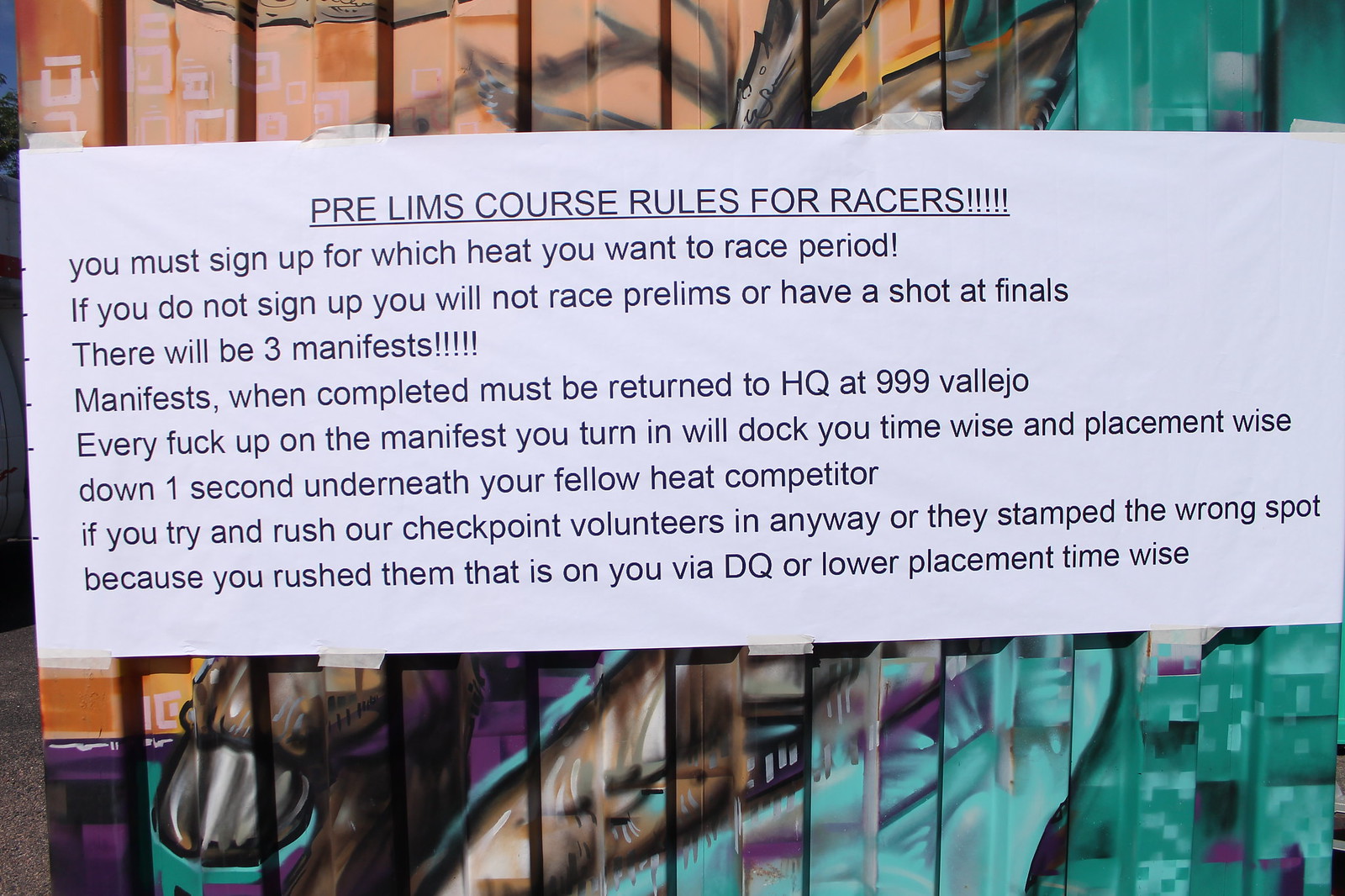The photo features a small, rectangular piece of white paper taped to what appears to be a storage container adorned with colorful graffiti art, including shades of orange, turquoise, and brown. The paper bears the bold, underlined header "Prelims Course Rules for Racers" with several exclamation points for emphasis. The text underneath lays out crucial race instructions: racers must sign up for their preferred heat; failure to do so will disqualify them from both prelims and finals. It continues to explain that there will be three manifests, and upon completion, these must be submitted to HQ at 999 Vallejo. Any mistakes on the manifests will result in a time penalty, deducting one second per error from the racer's standing relative to their competitors. Furthermore, racers are warned not to rush checkpoint volunteers; if a volunteer stamps the wrong spot due to rushing, it will lead to disqualification or additional time penalties.